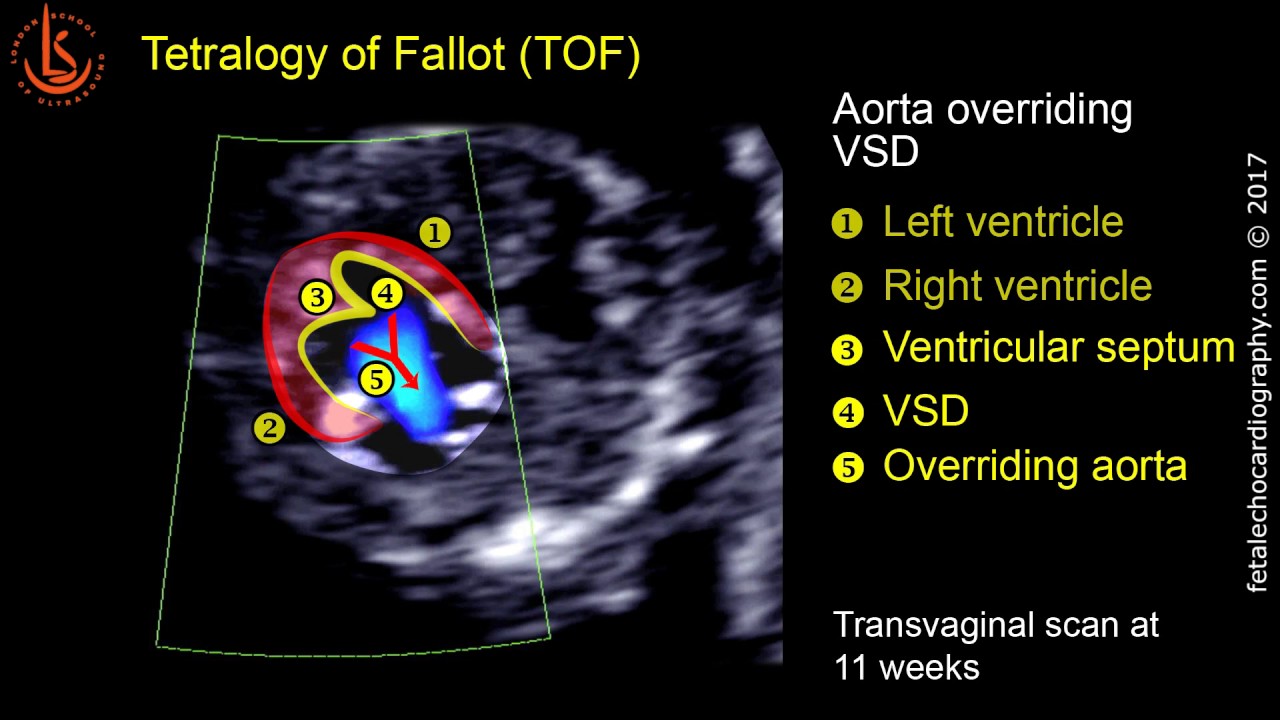This detailed image is a digitally-created ultrasound depicting Tetralogy of Fallot in a fetal heart at 11 weeks gestation, captured via transvaginal scan. The illustration features distinct colors including red, blue, yellow, black, off-white, white, and gray, creating a clear and informative visualization. Key anatomical structures are labeled with arrows and numbers (1 through 5), indicating the left ventricle, right ventricle, ventricular septum, ventricular septal defect (VSD), and an overriding aorta. The image is marked with the text "Tetralogy of Fallot," "TOF," and includes details such as "aorta overriding VSD," emphasizing the congenital heart defect. The layout positions the aortic and valvular details to the left, while the text annotations are placed on the right and top-left sections of the image. The image includes references to "fetal shawcardiography.com," copyright 2017, and features URLs such as www.ottobock.com.